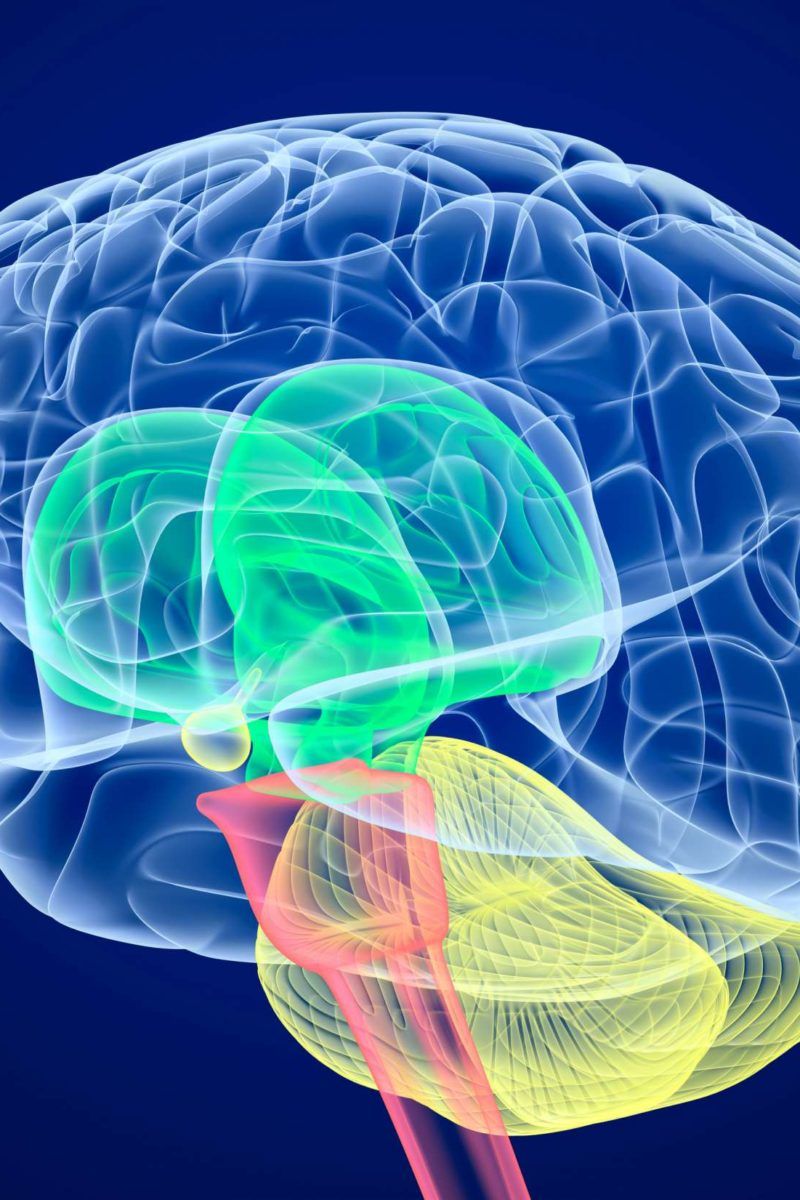The digital image showcases a CGI-rendered human brain against a dark blue backdrop. The primary brain structure is illustrated in a semi-transparent white, complete with detailed grooves that mimic those of a real brain. Within this translucent white brain, various regions are highlighted in distinct colors: the spinal cord is represented in red, two central areas are marked in neon green, and an additional lower area is depicted in neon yellow. All these colored regions are also semi-transparent and appear layered within the main brain structure, creating a multi-dimensional effect. This meticulous rendering emphasizes the complex anatomy and connectivity of the human brain through precise and distinguishable color-coding.